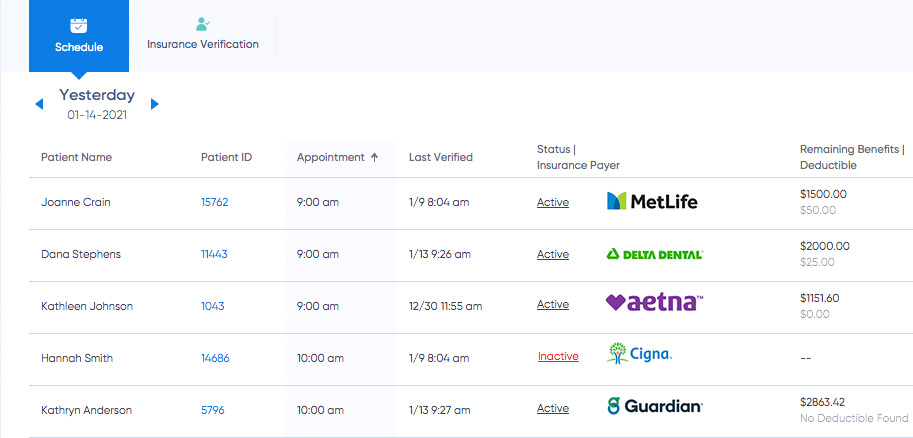A cropped screenshot of a doctor's office software interface is displayed. At the very top, a grey bar features the word "Schedule" on the left, accompanied by a blue box labeled "Insurance Verification." Below this bar, the interface shows navigation options, including "Yesterday" in dark grey font and the current date in small grey font, with arrows on either side to scroll through different days.

Further down, the layout includes a vertical column on the left listing patient names, followed by columns for patient ID, appointment time, last verification, status, insurance payer, remaining benefits, and deductible amounts. 

The first entry is for Joanne Crane. Her patient ID is displayed in blue, alongside her appointment time of 9 AM. Her last verification is logged at 19804 AM. Under the status column, she is marked as "Active." The insurance payer is MetLife, with the MetLife logo visibly to the right. Joanne's remaining benefits amount to $1,500, and her deductible is $50.

Each of the four other patient entries follows the same format, listing names on the left with corresponding patient IDs, appointment times, last verification times, statuses, insurance companies, and the remaining benefits and deductible amounts. The detailed information provides a comprehensive snapshot of patient schedules and insurance verifications for the day.